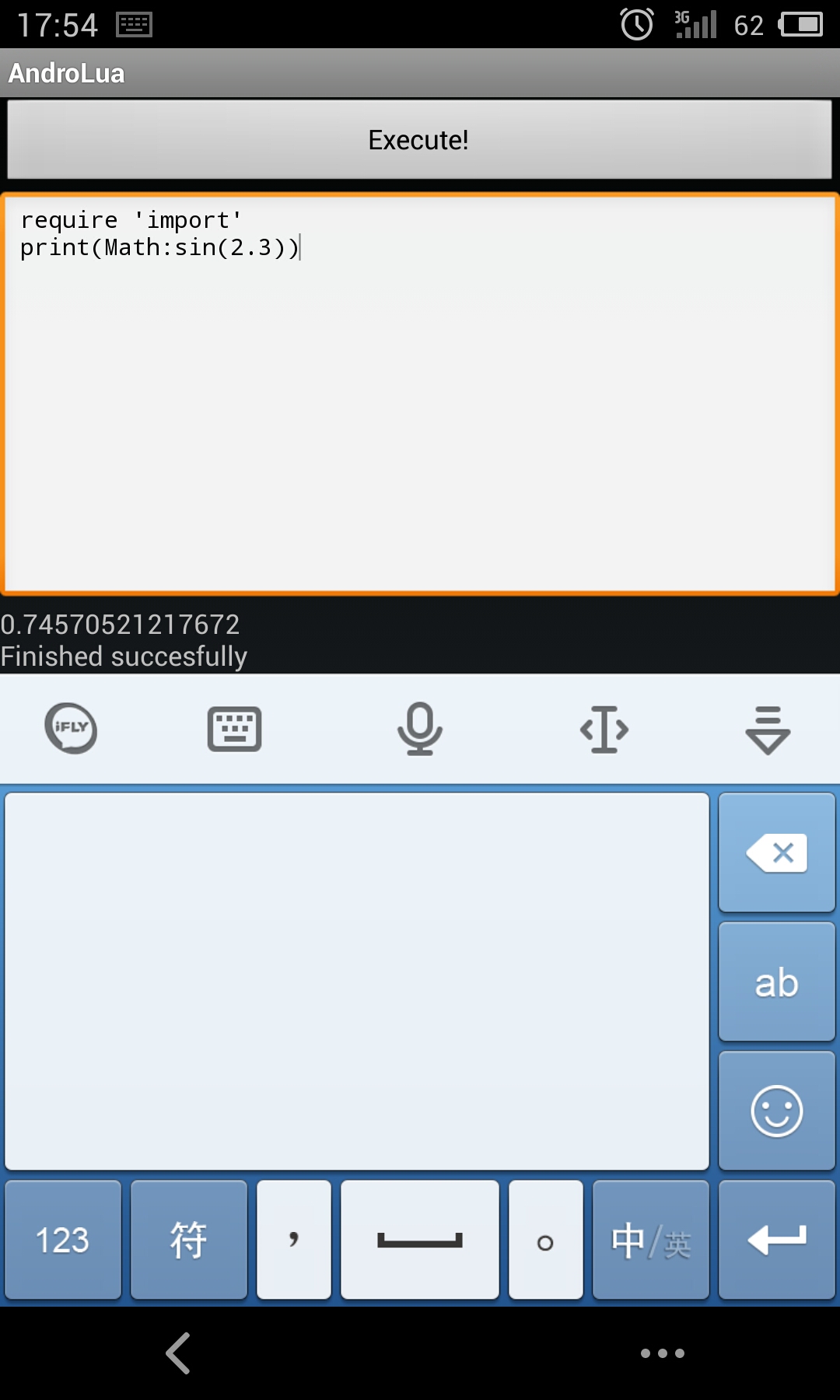A detailed screenshot of a smartphone interface is depicted. At the top left corner of the screen, within a long horizontal black rectangle, the time is displayed as "1754" in grey text. Adjacent to the time, a grey icon resembling a keyboard is visible. On the far right side, the status bar includes a sequence of icons: a clock, a bar graph representing the data signal, the number "62", and a battery icon indicating that it is 62% charged. 

Just below the status bar, a grey horizontal bar with white text reads "Andro Lua". Beneath this bar, a grey rectangle with black text centered within displays the word "Execute!" 

Further down, there is a grey box outlined in orange that contains programming script: "Require Import Print C Math: sin 2.3 print c print c ." Below this code, the text "finished successfully" appears in black, enclosed within grey text. 

At the bottom section, a blue horizontal bar displays five grey icons. Appearing underneath this bar is an interface similar to a calculator screen.